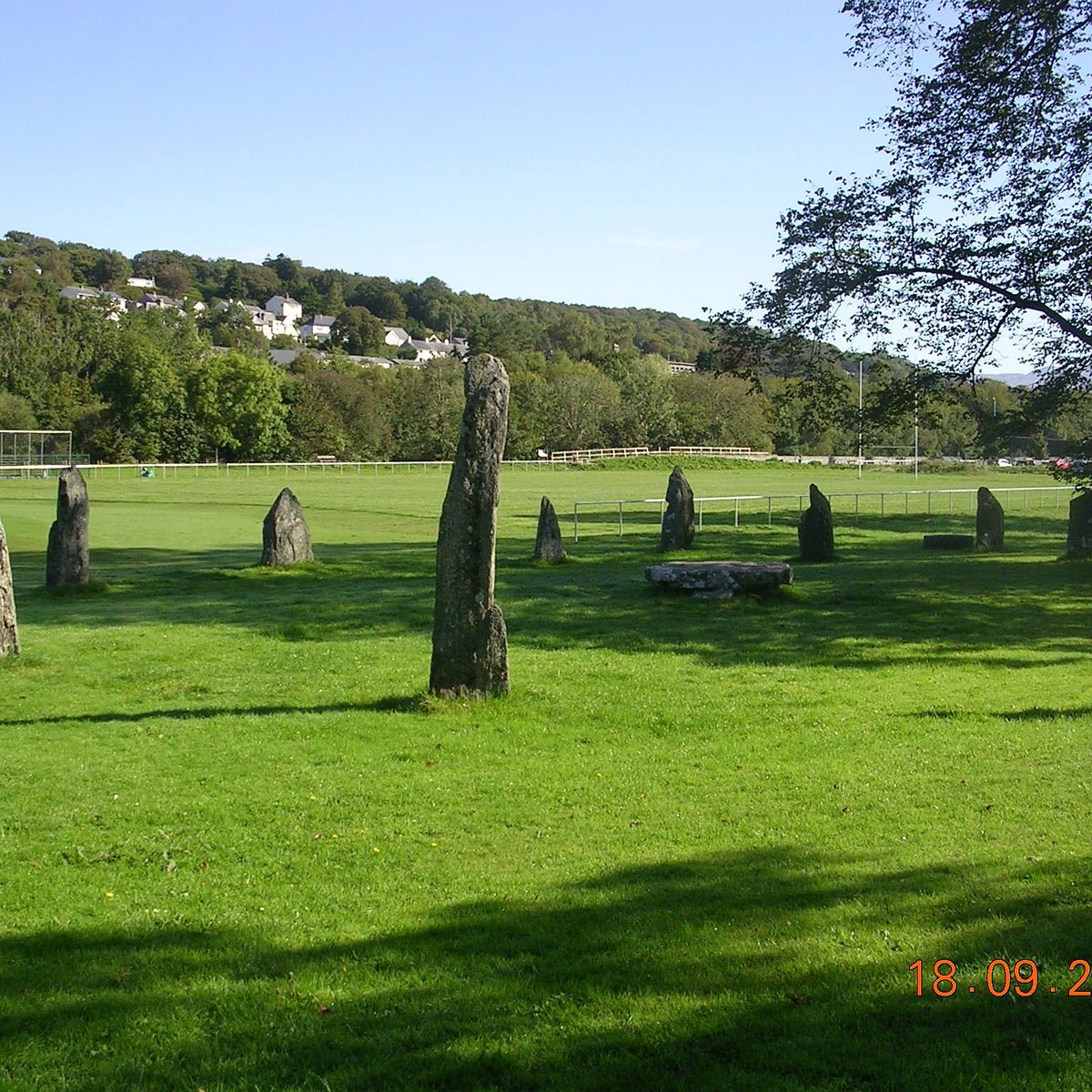The photograph captures a serene park landscape, featuring a striking stone circle arrangement. In the center of the image stands a tall, rounded stone, encircled by several shorter, jagged stones that form an uneven ring. A flat stone, resembling a bench, lies slightly offset from the central stone. The park's neatly maintained, flat green grass extends across the foreground, giving way to a gently sloping hill in the distance, adorned with small white and gray houses interspersed among lush trees. On the right side of the image, a large tree frames the scene, its branches partially visible, while further along the horizon, additional trees add depth to the vista. The sky above is a clear, light blue, suggesting a bright, sunlit day likely in spring or summer. Notably, the image contains a date stamp in the lower right corner, partially visible as "18.09.2," hinting at when this tranquil moment was captured.